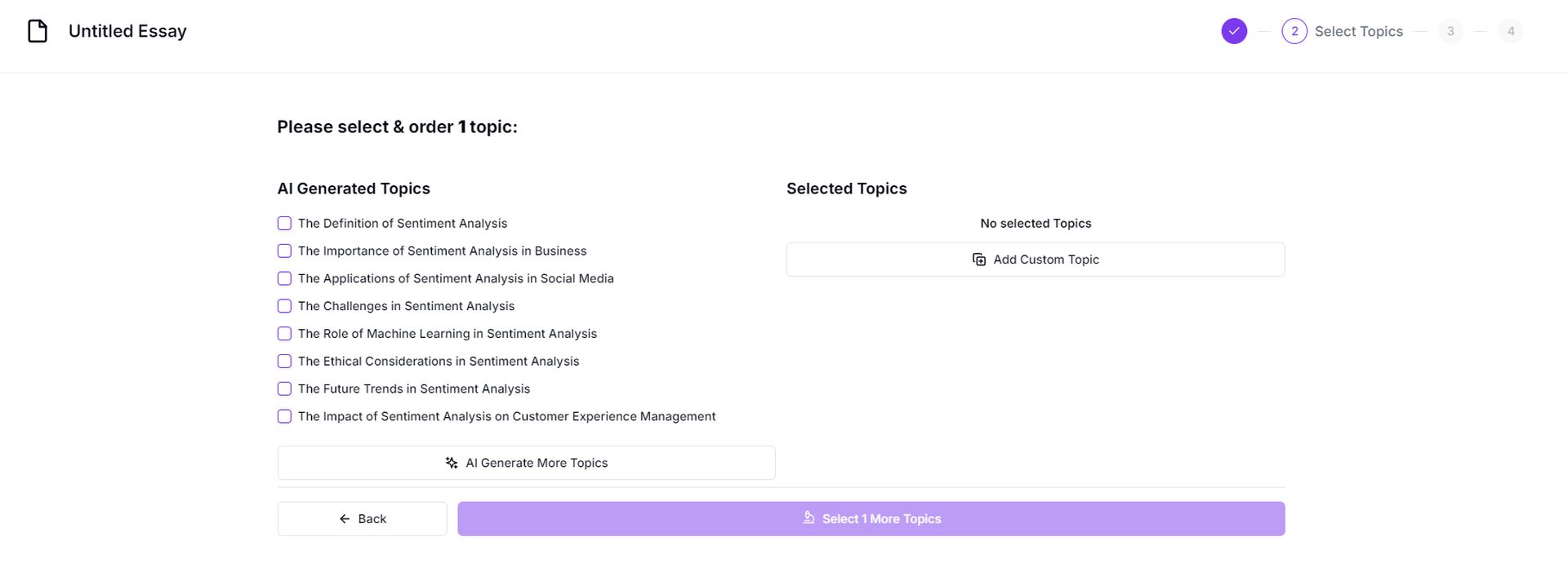Screenshot of a web page displaying the step-by-step process of creating an essay using an AI-generated tool. In the top left corner, the title "Untitled Essay" is visible, while the top right corner shows the label "Step 2." The current step, "Select Topics," is highlighted with a check mark on the left. Steps 3 and 4 are indicated but not yet selected.

Below the heading are instructions prompting the user to "Please select or order one topic." The section titled "AI Generated Topics" lists about a dozen topics, each accompanied by a checkbox. Example topics include "The Definition of Sentiment Analysis" and "The Importance of Sentiment Analysis in Business."

Underneath the topic list, options are available for viewing "No Selected Topics" or adding "Custom Topics." At the very bottom of the page, navigation buttons are provided: a "Back" button on the left and a purple, rectangular button on the right labeled "Select One or More Topics."

The user is in the middle of refining their essay structure and has not yet selected any topics from the list.